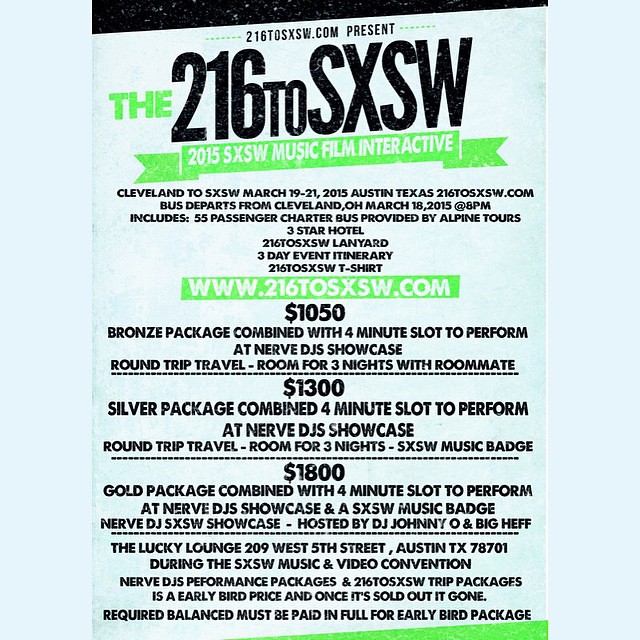The image is a detailed poster advertising the 216 to SXSW event. At the top, in black font, it reads "the 216 to SXSW," with a green banner beneath it displaying "2015 SXSW Music Film Interactive" in white font. Below, in black font, the poster states "Cleveland to SXSW, March 19-21, 2015, Austin, Texas" and provides the website "216TOSXSW.com." Further details include a bus departing from Cleveland, Ohio, on March 18, 2015, at 8 pm, with transportation being a 55-passenger charter bus provided by Alpine Tours. Accommodation includes a 3-star hotel and a 3-day event itinerary, along with a 216TOSXSW t-shirt. 

The packages available are outlined next: 
- The bronze package, costing $1,050, includes a 4-minute slot to perform at the NERV DJ Showcase, round-trip travel, and a room for 3 nights.
- The silver package, priced at $1,300, offers similar benefits with an SXSW music badge.
- The grand package, costing $1,800, includes a 4-minute performance slot, an SXSW music badge, and additional features hosted by DJ Johnny O and Big Hef.

Finally, it mentions the event location, The Lucky Lounge, at 209 West 5th Street, Austin, TX 78701, and emphasizes that there are early bird prices which must be paid in full once sold out.